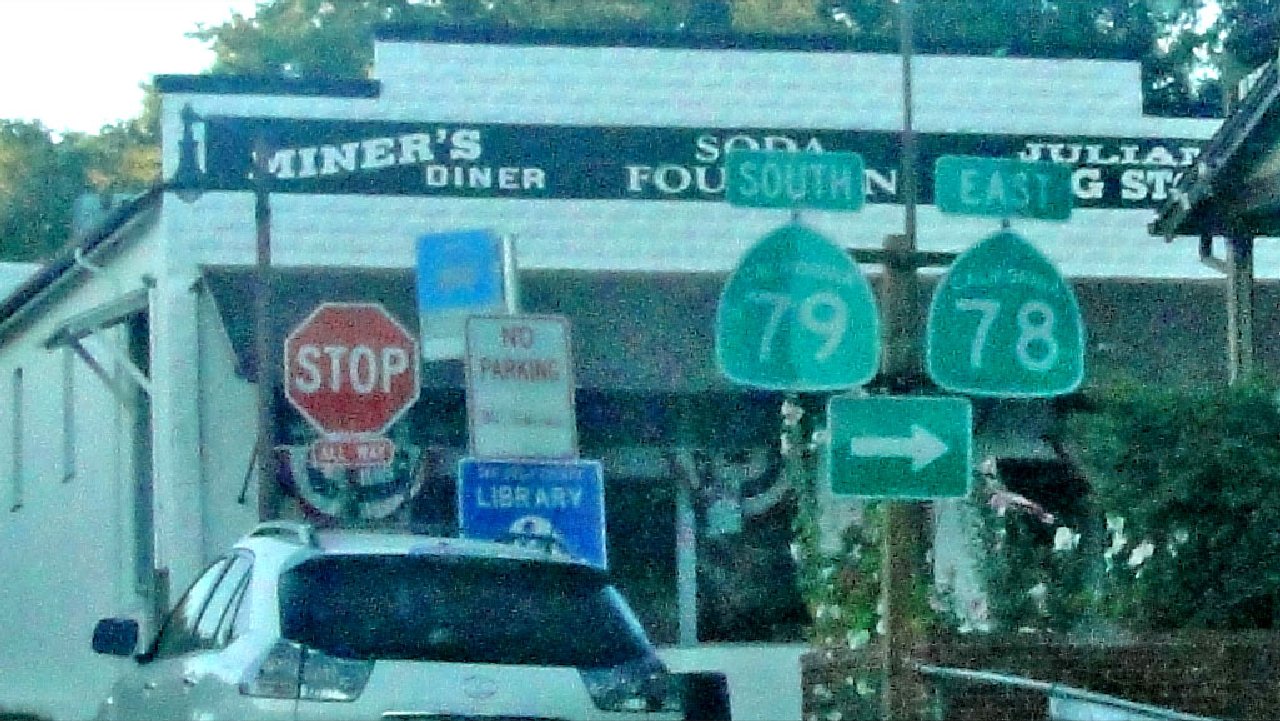This color photograph, although grainy and slightly desaturated, evokes a nostalgic, vintage feel, as if captured on film or with a retro filter. Dominating the bottom left corner are multiple road signs, which provide a focal point of interest. The centerpiece of the image is the back of a silver car, parked with an air of timelessness.

Above the car, the scene is framed by a cluster of green-leaved trees standing partially in front of a bridge or building to which some of the signs are attached. The building in the background, constructed from white bricks, prominently features a dark sign with white lettering that reads "Miner's Diner." Just beneath it, partially obscured by a road sign, are the words "Social Soda Fountain," harkening back to a bygone era.

In the upper-left corner of the photograph, the sky is overexposed to a stark white, contrasting with the scene below. Below the white sky, the visual narrative continues with several signs: a red stop sign prominently positioned in front of the car, a "No Parking" sign rendered in white, and a sign that could possibly say "Library," albeit it's challenging to decipher.

Flanking the initial set of signs, further to the right, are additional green road signs: one indicating "South 79," another "East 78," and a third sign beneath them with an arrow pointing to the right. The tableau is completed with more trees clustered at the lower right, adding a touch of natural greenery to the urban scenery.